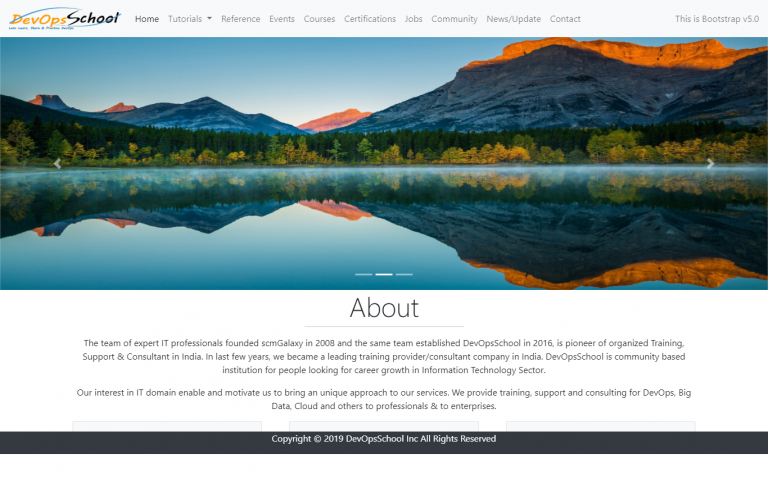**Image Caption:**

In the upper left corner of the image, the name "DevOps School" is prominently displayed. The word "DevOps" is in vibrant yellow, while "School" is in black, all set against a clean white background. On the right side of the "DevOps School" text, there are several navigation tabs written in black, arranged from left to right: Home, Tutorials, Reference, Events, Courses, Certifications, Jobs, Community, News/Updates, and Contact. The top right corner of the image features a note stating "This is Bootstrap v5.0."

The center of the image showcases a serene landscape. A tranquil blue lake occupies the bottom portion, perfectly mirroring the scenic surroundings. Above the lake, lush green trees, some tinged with yellow, are situated. Further back, the landscape is adorned with mountains that have a brownish hue, partially covered in shadow, which are also reflected in the still waters of the lake.

At the bottom of the image, there is a text section titled "About." It narrates the history of DevOps School, highlighting that a team of expert IT professionals founded SCM Galaxy in 2008, and subsequently established DevOps School in 2016. Described as a pioneer in providing organized training, support, and consulting services in India, DevOps School has evolved into a leading training provider and consulting company in recent years. The institution is community-based, aimed at individuals seeking career growth in the IT sector, and it prides itself on a unique approach to its services. The school offers training, support, and consulting in areas such as DevOps, Big Data, and Cloud to both professionals and enterprises. The image concludes with a copyright notice at the bottom: "©2019 DevOps School Inc. All rights reserved."